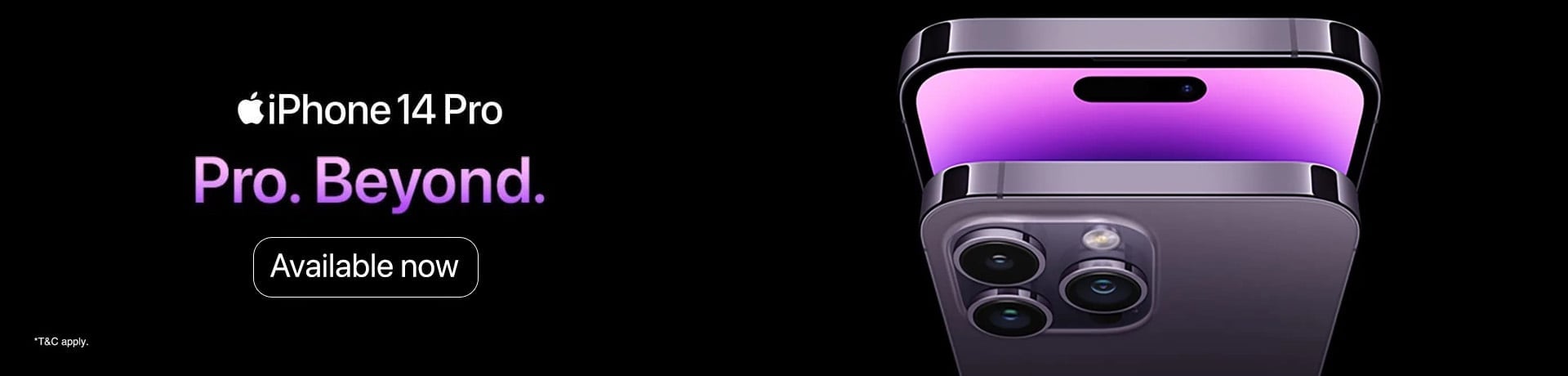This advertisement for the iPhone 14 Pro features a sleek and sophisticated design on a horizontal black background. The left side showcases text and graphics promoting the phone, starting with the iconic Apple logo and the words "iPhone 14 Pro" in white. Below that, in larger, stylized text with a gradient from light to dark purple, it reads "Pro. Beyond." The gradient effect gives the text a dynamic look, transitioning from a lighter shade at the top to a deeper purple at the bottom. Beneath this phrase, a black box with a white border and text announces "Available Now," likely serving as a hyperlink to the Apple website for purchasing the phone.

On the right side of the image, two iPhones are prominently displayed. The top phone is positioned slightly tilted to reveal a portion of its vibrant purple screen, which is turned on. The device showcases a sleek silver or aluminum finish, exuding a premium feel. The bottom phone is shown from the back, highlighting the advanced camera system with three lenses and a light, emphasizing the phone's cutting-edge photographic capabilities. This polished advertisement effectively captures the elegance and technological sophistication of the iPhone 14 Pro.